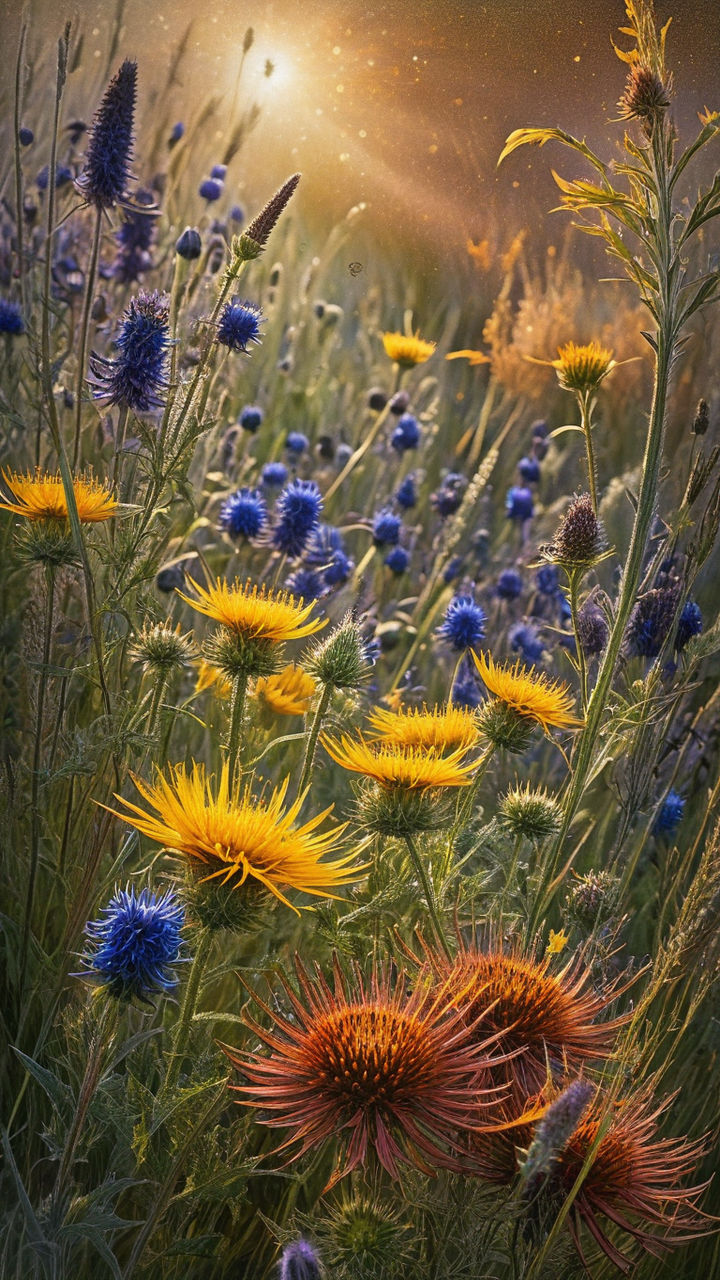The painting depicts a vividly detailed outdoor scene in portrait mode, featuring a lush field brimming with various types of flowers under a radiant sky. In the bottom right corner, three distinct globe-shaped, orange spiky flowers stand prominently. Interspersed across the field are clusters of yellow dandelions, characterized by their green stems and bright yellow petals, mingling with a series of oval-shaped blue flowers that stretch upwards. The top left corner showcases purple, cone-shaped flowers silhouetted against a dark, star-studded sky. In the top right, a majestic sunflower stands out against the celestial backdrop. The sky, though primarily black and dark, is illuminated by what appears to be either the sun or the moon, casting a warm glow over the scene, with hints of yellow adding a futuristic ambiance. The field is rendered with tall, high grasses, enhancing the natural, unkempt beauty of the landscape. The painting’s range of colors—from vivid greens and yellows to deep blues and oranges—highlights the rich diversity and clarity of this strikingly illuminated outdoor setting.